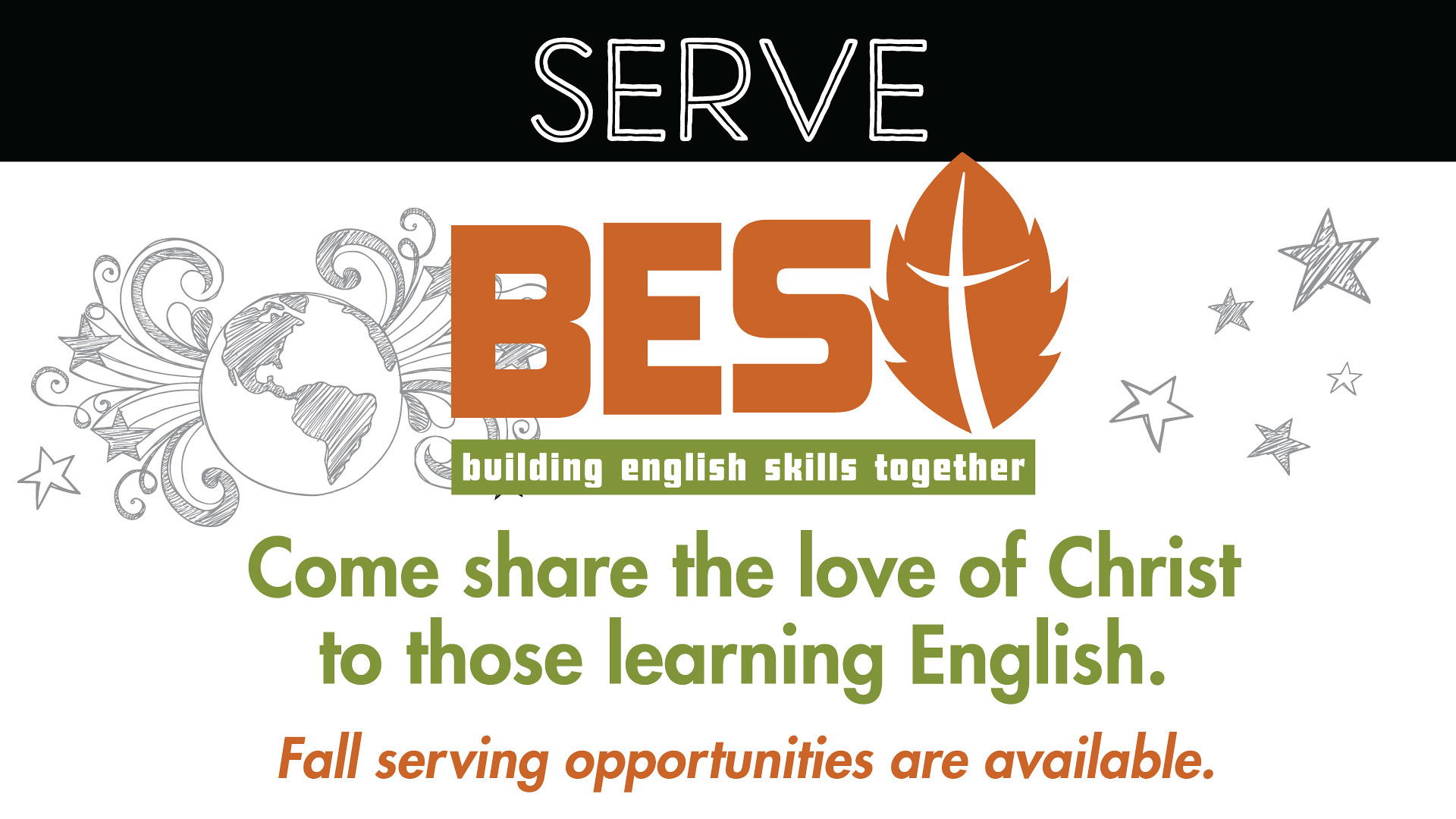This visual advertisement, which appears to be a business card or magazine banner, promotes a church event focused on community service and learning English. Set against a white background, the design features a distinctive black bar at the top, emblazoned with the word "SERVE" in white letters. Below this, a hand-drawn illustration of the Earth shows primarily North America, sketched in pencil-like lines, flanked by decorative elements and stars. Central to the design is a prominent logo with the text "BEST" in burnt orange; the "T" is uniquely designed as a white cross set against a burgundy and burnt orange leaf. Beneath the logo, a green banner with white text reads "BUILDING ENGLISH SKILLS TOGETHER." Further down, additional green text invites: "COME SHARE THE LOVE OF CHRIST TO THOSE LEARNING ENGLISH." The advertisement concludes with an announcement in burnt orange about available fall serving opportunities.